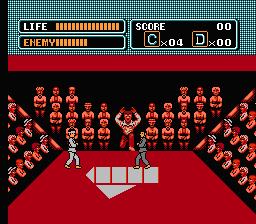This image is a nostalgic screenshot from a retro two-dimensional video game, showcasing a classic fighting scene. At the bottom of the screen, two characters are engaged in a combat match within a ring, surrounded by a vibrant crowd of spectators. In the center of the ring stands a referee with his hands raised, seemingly officiating the match. The character on the left is dressed in a traditional white karate suit, while the fighter on the right sports a light gray karate suit. Above the scene, a life bar for each fighter is displayed, alongside an enemy life bar, indicating the current health status of each character. To the right of the life bars, a score card is visible, labeled with the letters 'C' and 'D,' accompanied by various numbers, possibly representing points or other in-game statistics. This intricate scene captures the essence of retro gaming with its detailed pixel art and classic fighting game elements.